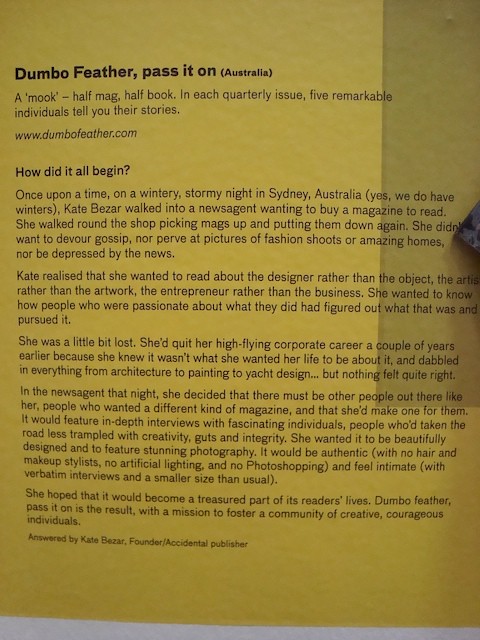The image depicts a yellowed page, possibly from a book, pamphlet, or scan, featuring black text with a slightly shadowed top edge. Dominating the top in large, bold font are the words: "DUMBO FEATHER, PASS IT ON, AUSTRALIA." Beneath this, a subtitle reads: "A MOOC, Half Mag, Half Book. In each quarterly issue, five remarkable individuals will tell you their stories." The web address "www.dumbofeather.com" is italicized below. The document's paragraph heading poses the question: "How Did It All Begin?"

The text unfolds a narrative: "Once upon a time on a wintry, stormy night in Sydney, Australia—yes, we do have winters—Kate Bazar walked into a newsagent wanting to buy a magazine to read. She wandered the shop, picking up magazines and putting them back down. She didn't want to devour gossip, gaze at fashion shoots or luxurious homes, nor be depressed by the news. Instead, Kate yearned to read about the person behind the design, the creator over the creation, the innovator over the innovation. This realization led to 'Dumbo Feather, Pass It On' with a mission to foster a community of creative, courageous individuals. Kate hoped it would become a cherished part of its readers' lives, thus resulting in DUMBO FEATHER, PASS IT ON, answered by Kate Bazar, founder and accidental publisher."